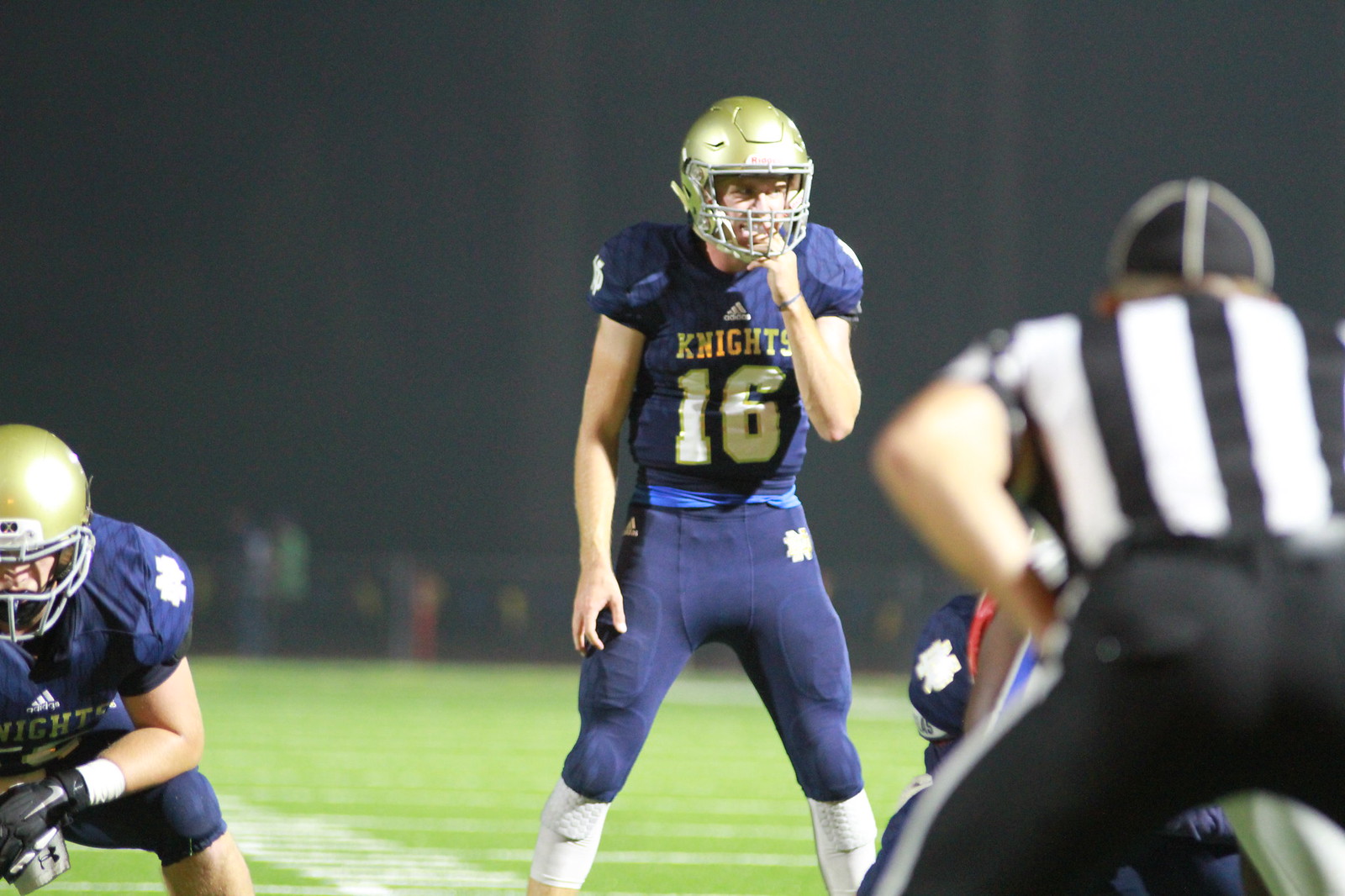This action photograph captures an intense moment of a night football game featuring the Knights. Set against the black sky illuminated by stadium lights, the image highlights the green field and players poised for action. In the center, the quarterback, adorned in a navy blue jersey with "16" and a gold helmet, is adjusting his mouthpiece, signaling his readiness to call a play. His uniform reads "Knights" on the front. Flanking him are two offensive linemen; one to the right in a partial squat, and the other’s shoulder is visible on the left. The scene suggests a high-stakes situation, possibly near the goal line, poised to score. In the foreground, an out-of-focus referee in a black-and-white striped shirt and black pants is squatting, focused intently on the impending play, with his back to the camera. The background features blurry figures standing behind a fence, adding to the anticipation of the moment about to unfold in this exciting football match.